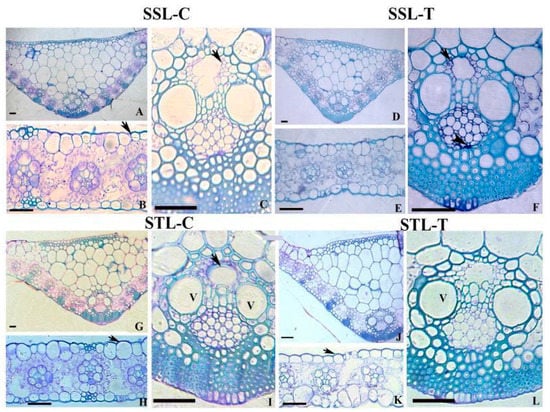This image is a detailed scientific illustration showcasing a series of stained cellular materials viewed under a microscope. The illustration is divided into four quadrants, each labeled with specific abbreviations: SSL/C (top left), SSL/T (top right), STL/C (bottom left), and STL/T (bottom right). The images feature clusters of circles and bubbles in a pastel color palette dominated by blues, pinks, and purples, set against light backgrounds of white or light yellow. Each quadrant contains several smaller images enumerated with letters from A to L, indicating distinct sections within each category. The overall visual effect is somewhat artistic, with concentric and aggregated circles of varying sizes that look almost like artwork but depict scientific observations of cellular processes, possibly apoptosis. Some of the images show darker or more fragmented areas, suggesting variations in cellular structures.